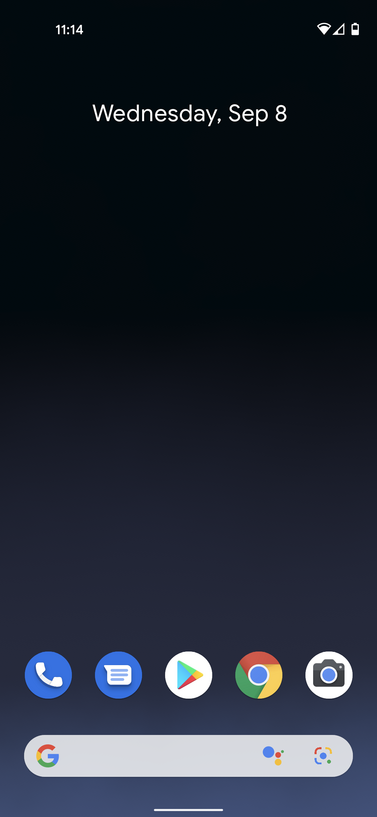The image displays a smartphone's home screen with various elements and applications.

- **Top Bar:** 
  - **Top Left Corner:** The time is displayed as 11:14 AM in white text.
  - **Top Right Corner:** Icons for Wi-Fi, network connection, and battery status (nearly half full), all in white.

- **Center:** 
  - The date "Wednesday, September 8th" is centrally positioned and gradually sliding upward. The date text is white.
  
- **Wallpaper:** 
  - The background of the home screen transitions from black at the top to purple at the bottom, blending together in the center.

- **Bottom Section Icons (from left to right):** 
  - **Phone Icon:** Blue and white
  - **Messaging App Icon:** Blue and white
  - **Google Play Store Icon:** A white rectangle oriented to the right with four colors: blue, yellow, green, and red
  - **Chrome Icon:** A circle containing the same four colors as the Play Store icon
  - **Camera Icon:** Incorporates white, black, and blue

- **Bottom Search Box:** 
  - Contains Google's search box with a white background
  - The "G" in "Google" features colors blue, red, yellow, and green
  - The Google Assistant icon has circles in blue, red, yellow, and green
  - The Google Lens icon resembles a camera lens and also uses the same Google colors

This detailed description captures the visual layout and color scheme of the smartphone's home screen, ensuring clarity for readers without access to the image.